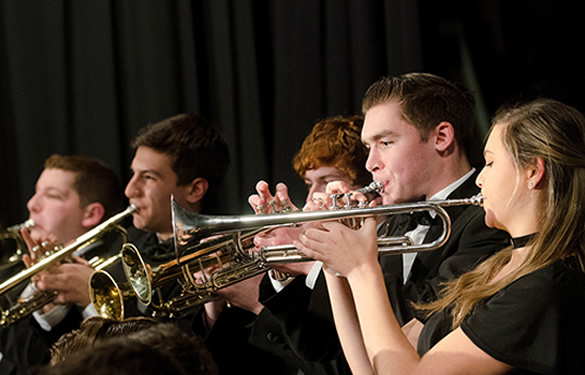In this image, we see five young adults, possibly high school students, performing on stage against a backdrop of black curtains. They are arranged in a row, each playing a polished silver trumpet. Starting from the left, the first musician is a girl with long, blonde hair, wearing a black dress and a black choker necklace. She holds her trumpet to her lips, fingers pressing on the first valve. Next to her is a young man in a black tuxedo with slicked-back hair, also actively playing his trumpet. Following him is another young man, distinguished by his orange hair, though his face is less visible. The fourth musician is slightly taller with dark black hair, and despite being a bit blurred, is similarly focused on playing his trumpet. The last player, also somewhat blurred, is another young man, completing the line of performers. All of them are intent on their instruments, creating a cohesive image of a synchronized trumpet section.